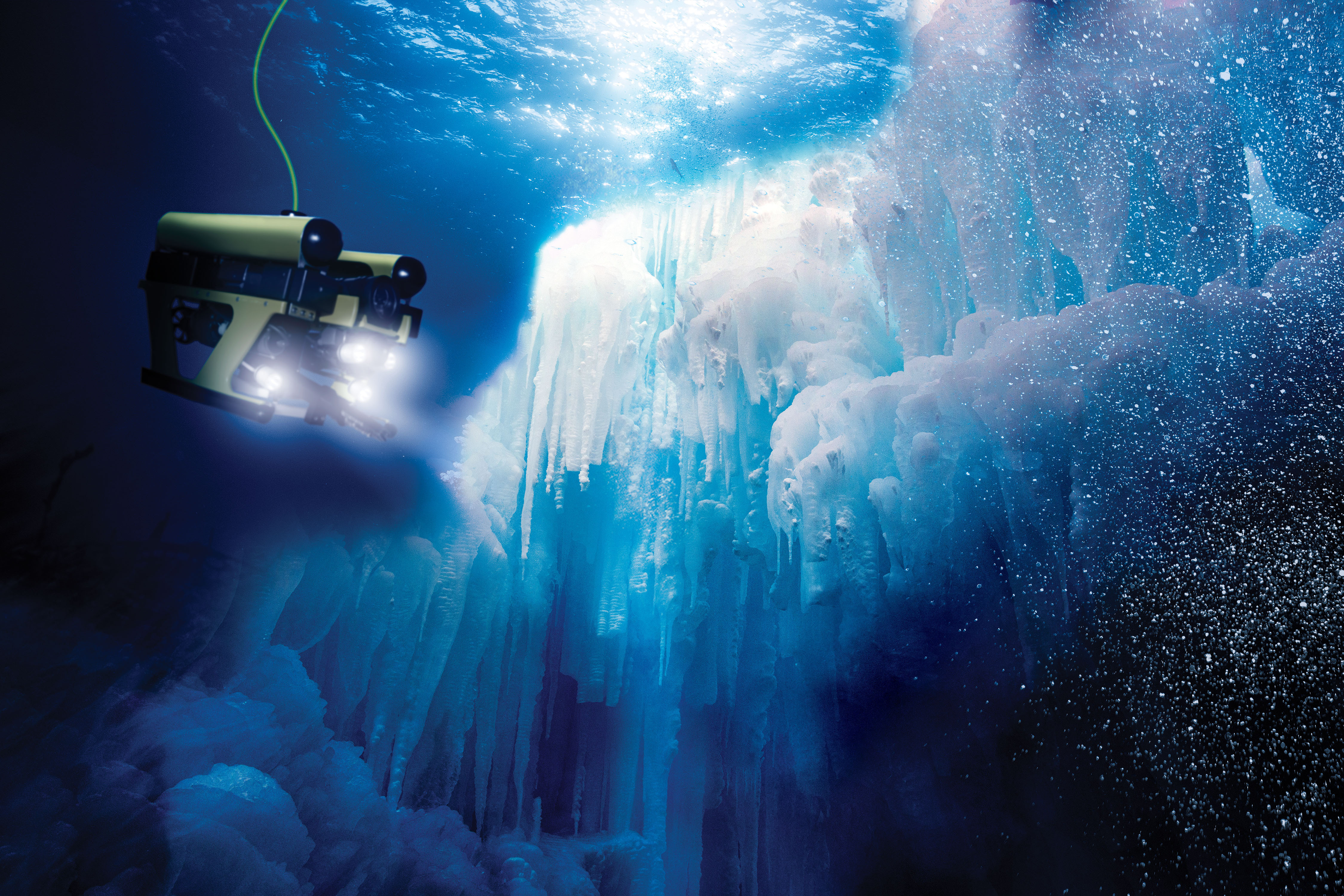The image depicts an underwater scene featuring a yellow submarine with black parts, navigating deep, frigid waters. The submarine, possibly a submersible camera, has two bright white lights on its lower section and a propeller at the back. It’s tethered to the surface by a green cord, likely an electrical line, which trails upwards towards light filtering through the water. Surrounding the submarine are massive chunks of ice and numerous spiky ice formations resembling underwater stalactites. On the right side of the image, bubbles rise from the depths, adding to the dynamic and detailed underwater atmosphere. The overall impression is so vivid and pristine that it creates an almost surreal, computer-generated appearance.